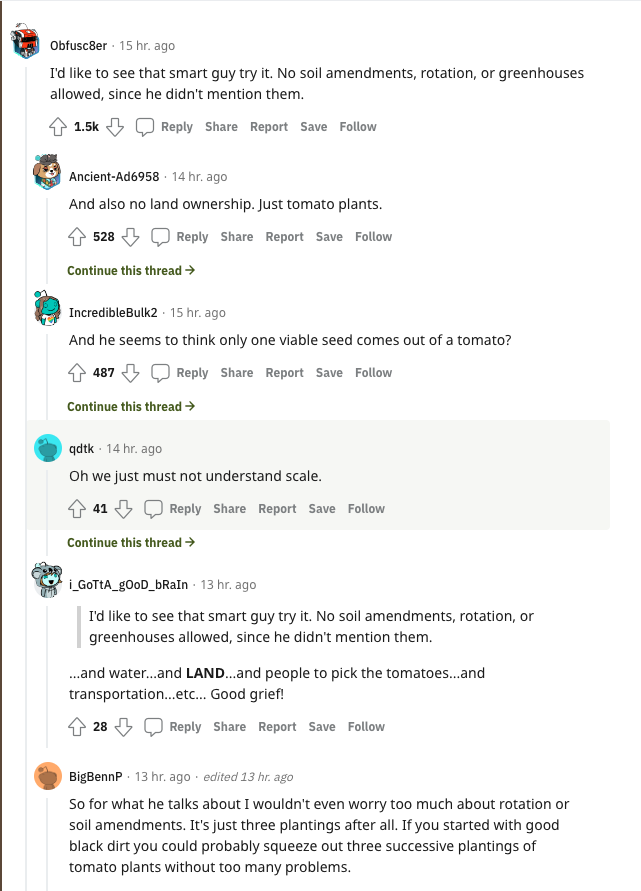**Reddit Discussion Detail: Tomato Planting Challenge Analysis**

**Screenshot Overview:**

Top Comment:
- **User:** Obsefusecar (Avatar: Semi-truck with a head)
- **Posted:** 15 hours ago
- **Comment:** "I'd like to see that smart guy try it. No soil amendments, rotation, or greenhouse allowed."
- **Engagement:** 1.5k upvotes
- **Options:** Reply, Share, Report, Save, Follow

Replies:
1. **User:** Ancient_add_6958
   - **Posted:** 14 hours ago
   - **Reply:** "And also no land ownership, just tomato plants."
   - **Engagement:** 528 upvotes
   - **Thread Option:** Continue this thread

2. **User:** Incredible_bulk_2
   - **Posted:** 15 hours ago
   - **Reply:** "And he seemed to think only one viable seed comes out of a tomato."
   - **Engagement:** 487 upvotes
   - **Thread Option:** Continue this thread

3. **User:** QDTK
   - **Posted:** 14 hours ago
   - **Reply:** "Oh, we just must not understand scale."
   - **Engagement:** 41 upvotes

4. **User:** I_got_a_good_brain (alternating capital and lowercase letters)
   - **Posted:** 13 hours ago
   - **Reply:** "I'd like to see the smart guy try it. No soil amendments, rotation, or greenhouse allowed. Since he didn't mention them." [Quotes Obsefusecar]
   - **Additional Commentary:** Emphasized "Water, and land" in bold. "And people get to pick the tomatoes and transportation, etc. Good grief!"
   - **Engagement:** 28 upvotes

5. **User:** BigBenP
   - **Posted:** 13 hours ago (edited)
   - **Reply:** "So for what he talks about, I wouldn't even worry too much about rotation or soil amendments. It's just three plantings after all. If you start with good black dirt, you could probably squeeze out three successive plantings of tomato plants without too many problems."

**Summary:**
This Reddit thread is focused on discussing the feasibility and challenges of tomato planting under stringent conditions, excluding soil amendments, crop rotation, or greenhouses. The conversation features various perspectives on agricultural practices, seed viability, land ownership, and logistical aspects of tomato production. User engagement through upvotes and detailed replies reflects a strong interest in the practical and theoretical aspects of sustainable agriculture and the hypothetical challenge presented.